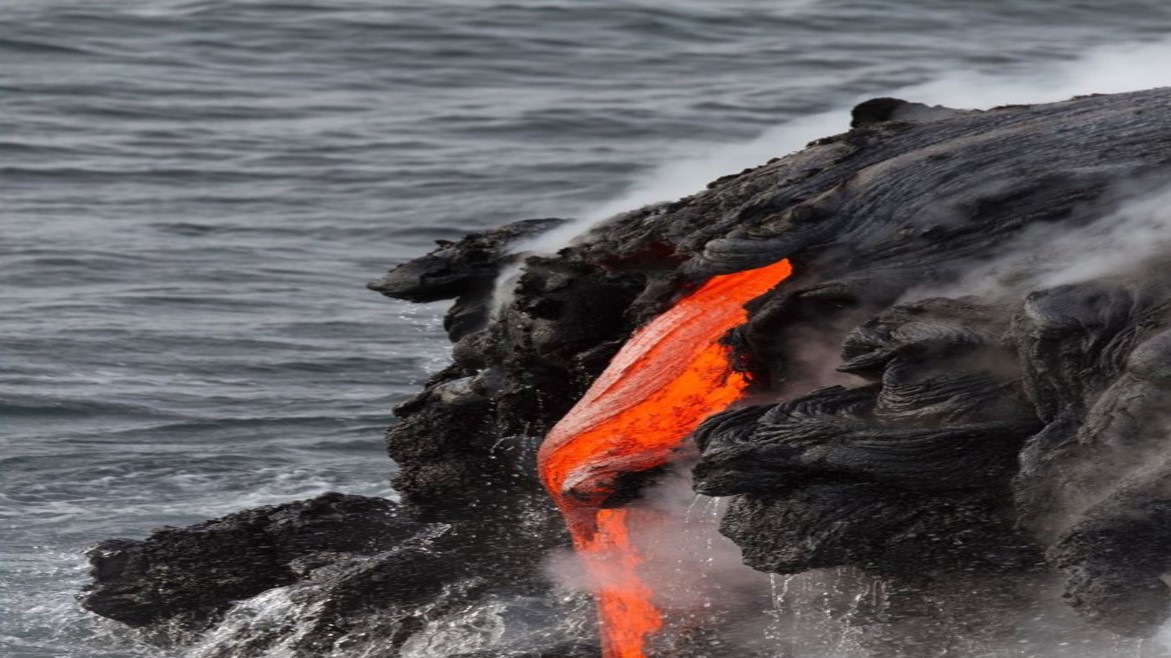The photograph captures a dramatic scene where bright red and orange lava emerges in a stream from a black rock formation on the right side of the image. The intense heat of the lava has formed new igneous rocks at its edges and is flowing directly into the dark blue, calm ocean visible in the background. Near the top of the rock formation, a plume of steam is seen rising and drifting to the right, staying low and close to the rocky surface. The edges of the cooling magma are covered with ash, adding to the stark contrast against the vibrant lava and the serene ocean backdrop. This ongoing volcanic activity hints at the continual creation of new landforms along this coastal setting.